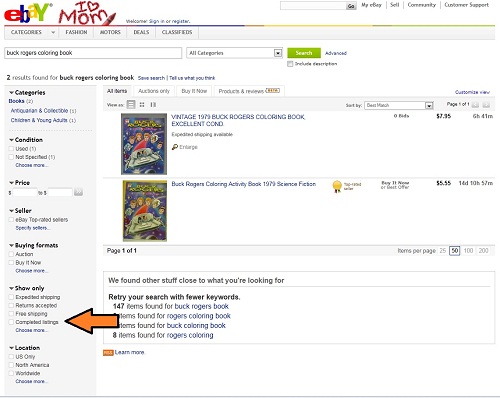Here is a cleaned-up and detailed description for the provided image:

---

This screenshot from eBay shows the homepage, prominently featuring the familiar eBay logo at the top left. Adjacent to the logo is a whimsical, childlike font inscription that reads, "I love mom." On the top right, a search bar is visible, accompanied by links labeled "My eBay," "Sell," "Comments," and "Customer Support."

Beneath this, a gray header displays navigational links including "Categories," "Fashion," "Motors," "Deals," and "Classifieds." Below the header, a search box is filled with the query "Buck Rogers Coloring Book," set to search in all categories, followed by a search button.

Two images of Buck Rogers coloring books are displayed, categorized by various criteria such as condition, price, seller, buying format, and location. The first listing is titled "Vintage 1975 Buck Rogers Coloring Book in excellent condition," priced at $7.95 with 6 hours and 41 minutes remaining on the auction. The second listing reads "Buck Rogers Coloring Activity Book 1979 Science Fiction," featuring an associated seller’s medal or award, priced at $5.56 with 1 day, 10 hours, and 52 minutes left.

At the bottom of the screenshot, a large rectangle offers related search suggestions under the text, "We found other stuff close to what you're looking for," followed by a prompt to "retry your search with fewer keywords." It mentions that 147 items were found for "Buck Rogers book," along with additional variations in the search results for "Rogers Coloring Book," "Buck Coloring Book," and "Rogers Coloring," though some of these numbers are partially obscured by an orange arrow pointing to the original gray column on the right. At the very bottom, there is a "learn more" link.